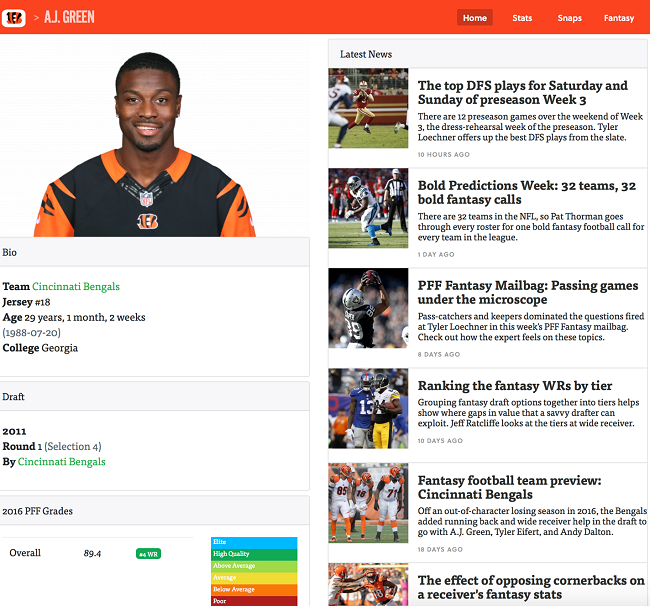Here's a cleaned-up and detailed caption for the described image:

---

This screenshot features the profile page of AJ Green on the Cincinnati Bengals' official website. The Bengals' logo is prominently displayed in the top right corner. The page is titled with AJ Green's name. Navigation tabs across the top offer sections for "Home," "Stats," "Snaps," and "Fantasy."

On the left side of the page, there is a striking image of AJ Green, a black man, wearing the Bengals' team uniform. The uniform's design includes a dark navy chest area complemented by orange sleeves and neckline. Emblazoned just below the neckline is the Bengals' logo, with the NFL logo positioned directly above it. Additional player details include:

- Name: AJ Green
- Team: Cincinnati Bengals
- Jersey Number: 18
- Age: 29 years, 1 month, 2 weeks
- Birth Date: July 20, 1988
- College: Georgia
- Draft Information: Drafted in 2011, Round 1, Selection 4 by the Bengals
- 2016 PFF Grades: Overall 89.4, Ranked #4 among wide receivers

To the right side of the page is a list of related news stories, including six articles with titles such as "Fantasy Football Team Preview" and "Bold Predictions for the Week."

---

This organized format provides a comprehensive and easy-to-read summary of the web page's content.